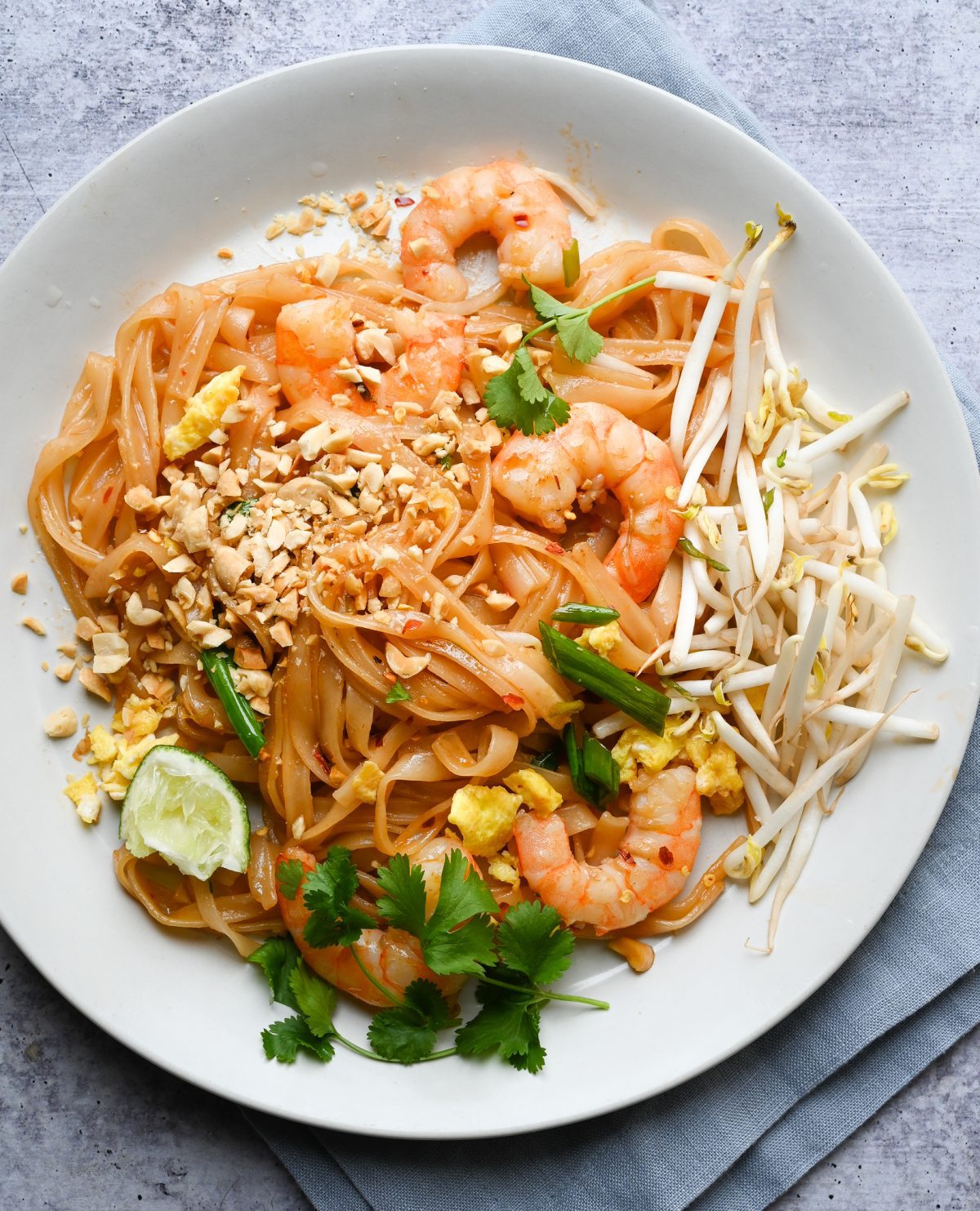The image showcases a beautifully arranged plate of Thai pad siew with shrimp on a white circular dish, placed on a gray cloth that sits atop a gray table. The dish features flat, light beige-pink noodles interspersed with several pieces of fried shrimp. There is a generous sprinkling of crushed peanuts over the noodles. Toward the bottom left of the plate rests a quarter wedge of lime, which appears to have been squeezed. Fresh cilantro serves as a garnish at the bottom of the dish, while crisp white bean sprouts are positioned on the right side. The vibrant elements come together to create a visually appealing, mouth-watering presentation.